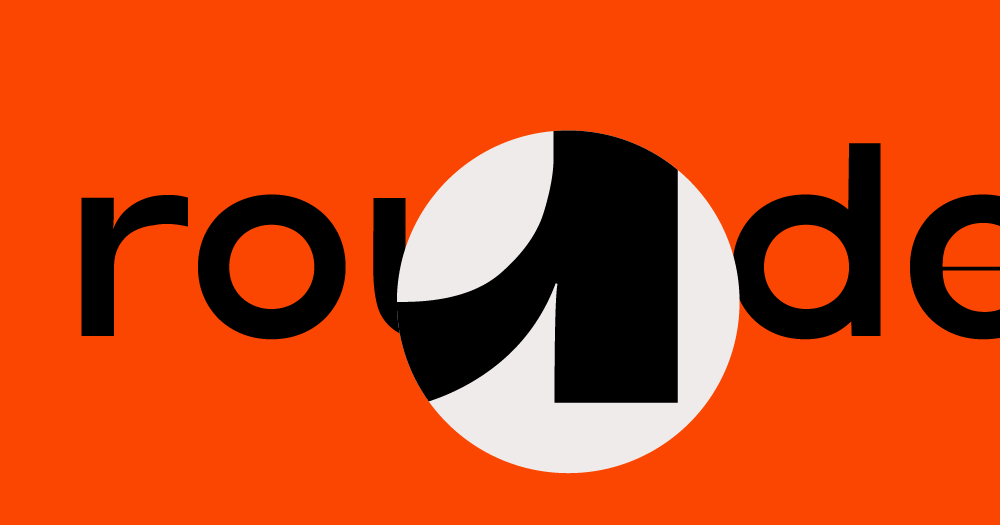The image depicts a rectangular space with a predominantly red or orange-red background, featuring black lowercase letters arranged to spell "roundo," although the word is not fully visible due to cropping. Centered on this background is a large white circle which acts as a magnifier, zooming in on the bottom part of the letter 'U'. The magnified view obscures the complete word, specifically covering up parts of the 'U' and 'D'. A black line runs horizontally through the entire image, intersecting the letters and the magnified circle, adding to the partial obscurity of the text. The overall composition emphasizes the fragmented view of the word through the interplay of colors and magnification.